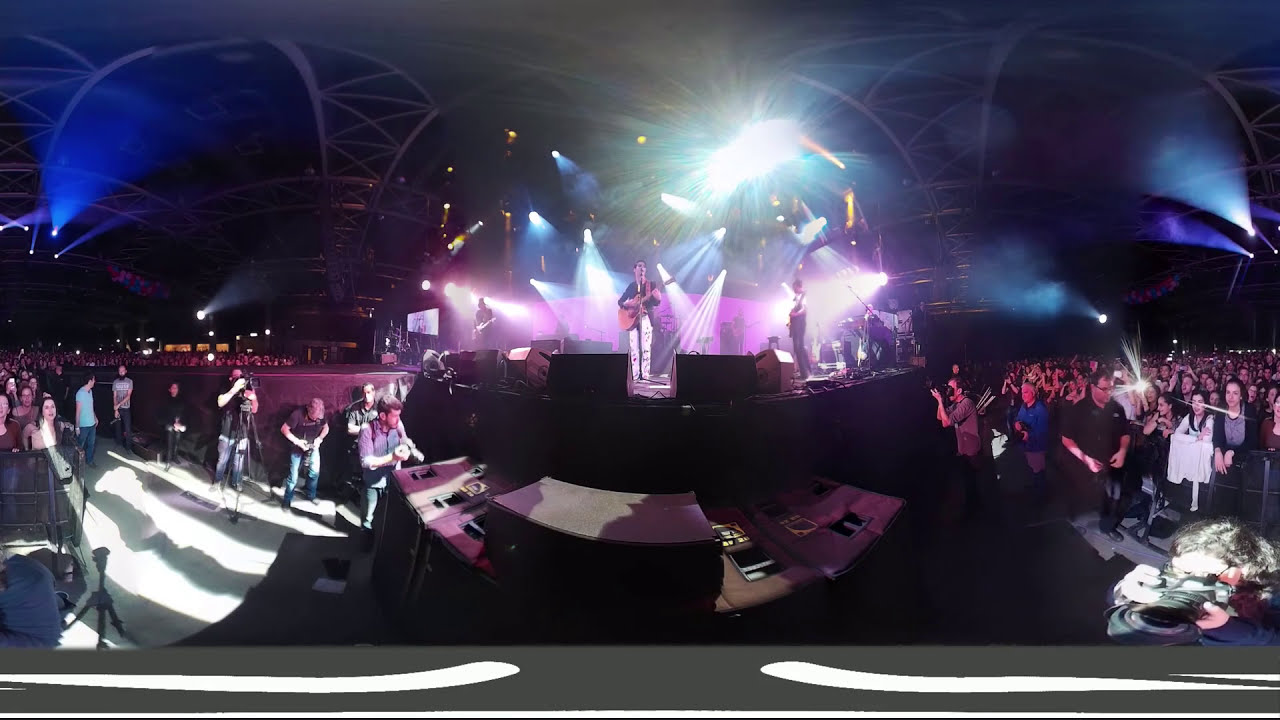In this vibrant panoramic photograph taken with a fisheye lens, a band is performing on a curved stage in the center of a dark indoor arena, dramatically lit by an array of bright, colorful lights in blues, purples, and greens, creating vivid streaks that cut through a haze of fog or smoke. The lead musician, easily noticeable in his white pants and blue top, stands at the forefront playing an acoustic guitar, flanked by band members in dark clothing. Shadows extend away from the stage due to the powerful violet spotlights behind them. To the left, cameramen aim their equipment at both the energetic crowd and the performers, capturing the electric atmosphere. The audience, dressed in a spectrum of colors, fills the stands primarily to the right of the stage, while some fans can be spotted toward the back left, adding to the sense of a packed venue. Above, a complex structure of curving support beams hosts additional lights that contribute to the vibrant and immersive environment, contrasting sharply with the surrounding arena's darkness. This entire scene is encapsulated in a single image, transforming the live concert experience into a wonderfully chaotic and colorful spectacle.